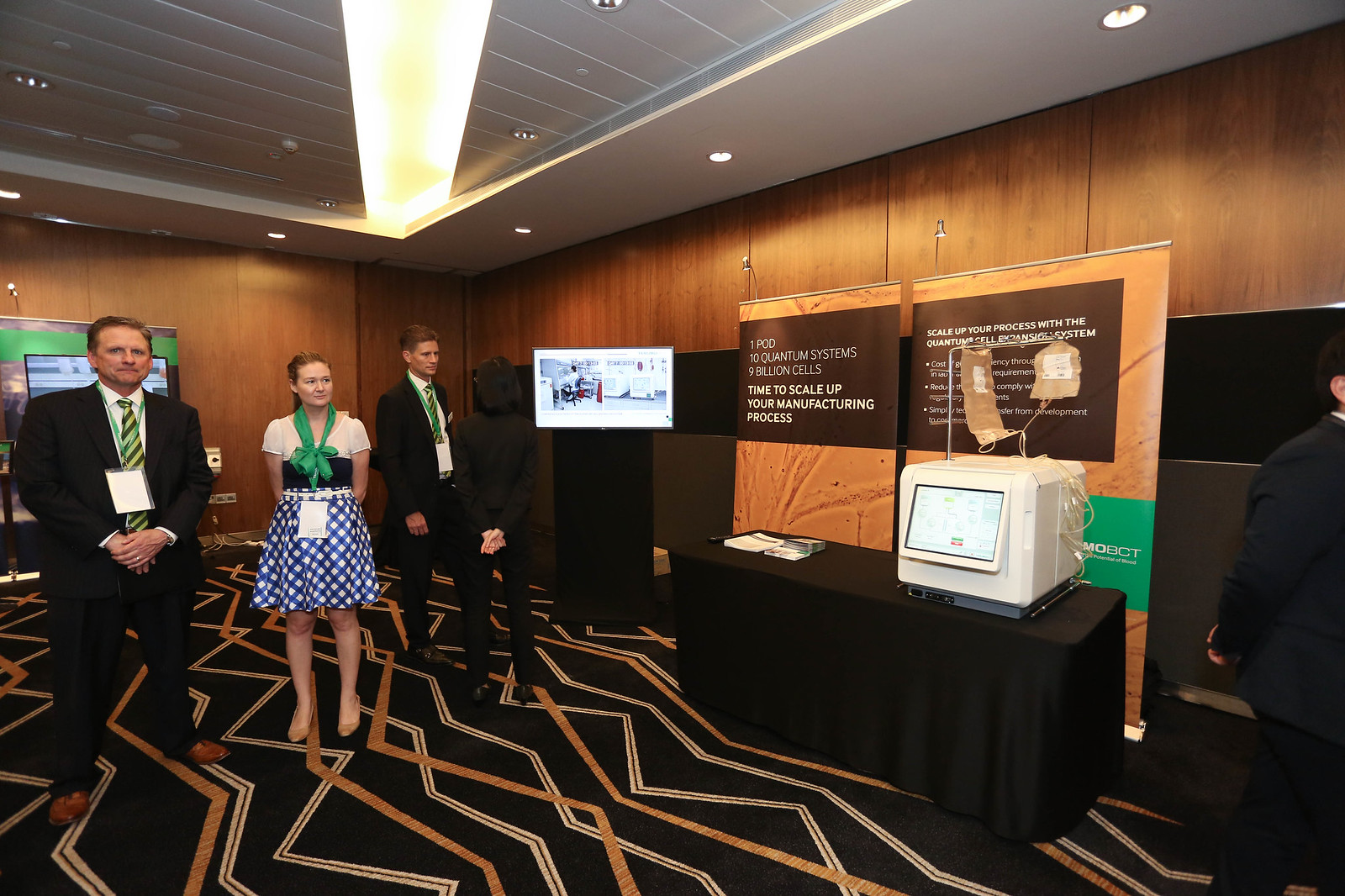The indoor photograph depicts a conference room with wooden paneled walls and a black carpet featuring zigzag designs in white, yellow, brown, and taupe. The ceiling is white with decorative lighting. There are multiple people in business attire standing in the room, with visible green lanyards. Positioned centrally is a young woman in a dress flanked by two men in suits, and another woman is facing away from the camera. On the right side of the image, there is a table draped with a black cloth, on which a white device resembling a computer with a display screen is placed. Behind this setup, two banners are visible, partially readable with text like "Time to scale up your manufacturing process," "Quantum Systems," and "Billion Cells." The overall scene evokes a professional and organized atmosphere, likely aimed at business or educational purposes.